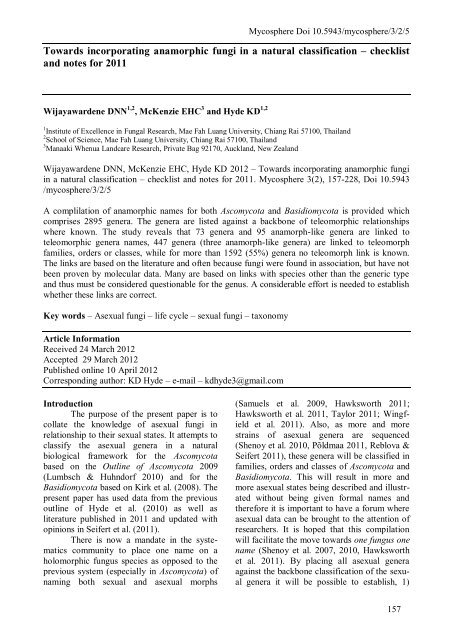The image depicts an excerpt from a scientific article titled "Towards Incorporating Anamorphic Fungi in a Natural Classification Checklist." This 2011 publication focuses on collating knowledge regarding asexual fungi and their relationship to sexual states. The document provides detailed information including the authors' names, keywords, and article information such as the corresponding author, K.D. Hyde (email: kdhyde3@gmail.com), and important dates: received on March 24, 2012, and published on April 10, 2012. The text appears in both English and another language, offering an introduction that states the paper's purpose and situates it within taxonomic research. The text spans page 157, and the entire image is in black and white without any images, presenting just a portion of the broader article.